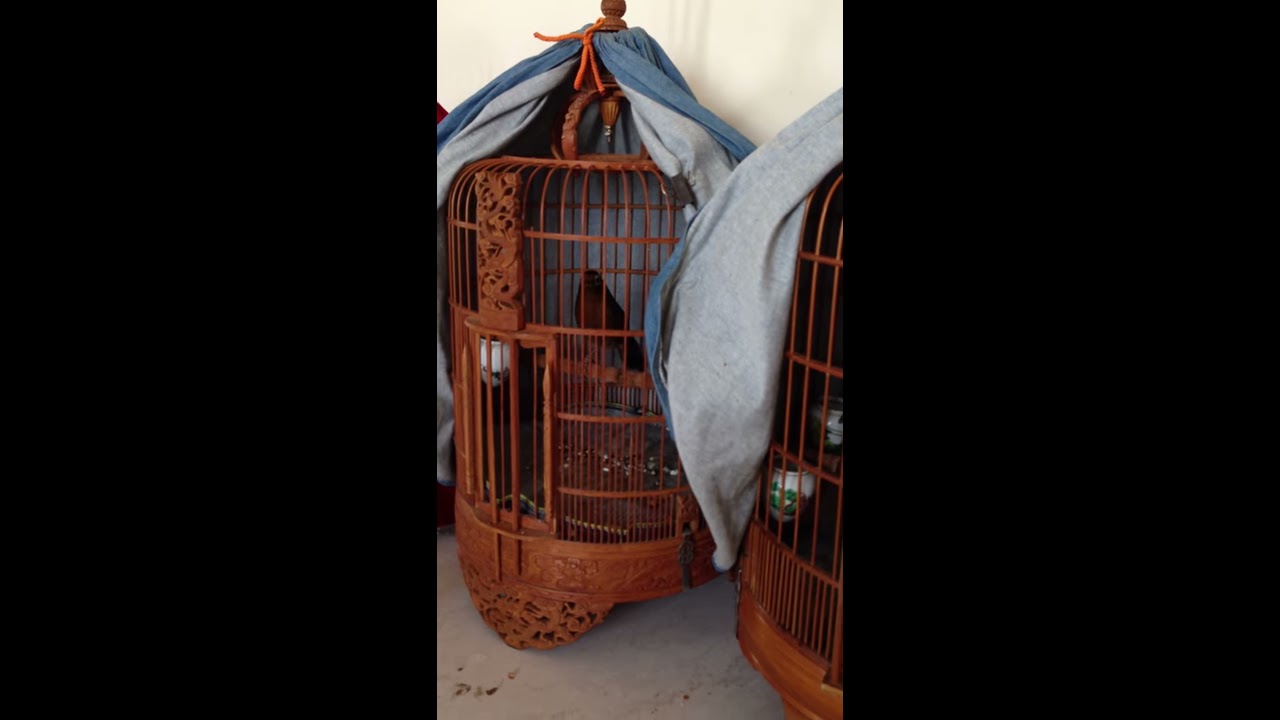The image features two elegant, brown wicker birdcages, each adorned with blue drapery on top. The primary birdcage is centrally positioned, showcasing intricate decorative designs and an orange-chested bird with a black back perched inside. This cage is partially covered, leaving the front open. A rope secures the cloth at the top. To the right, a second birdcage of identical design and drapery is only partially visible due to a black border framing the image. The setting appears to be a brightly lit room with white walls and a light gray cement floor. Inside the right-side birdcage, which appears less visible, there are teacups. The overall composition is framed by two black rectangular borders on either side, providing a classic, symmetrical layout.